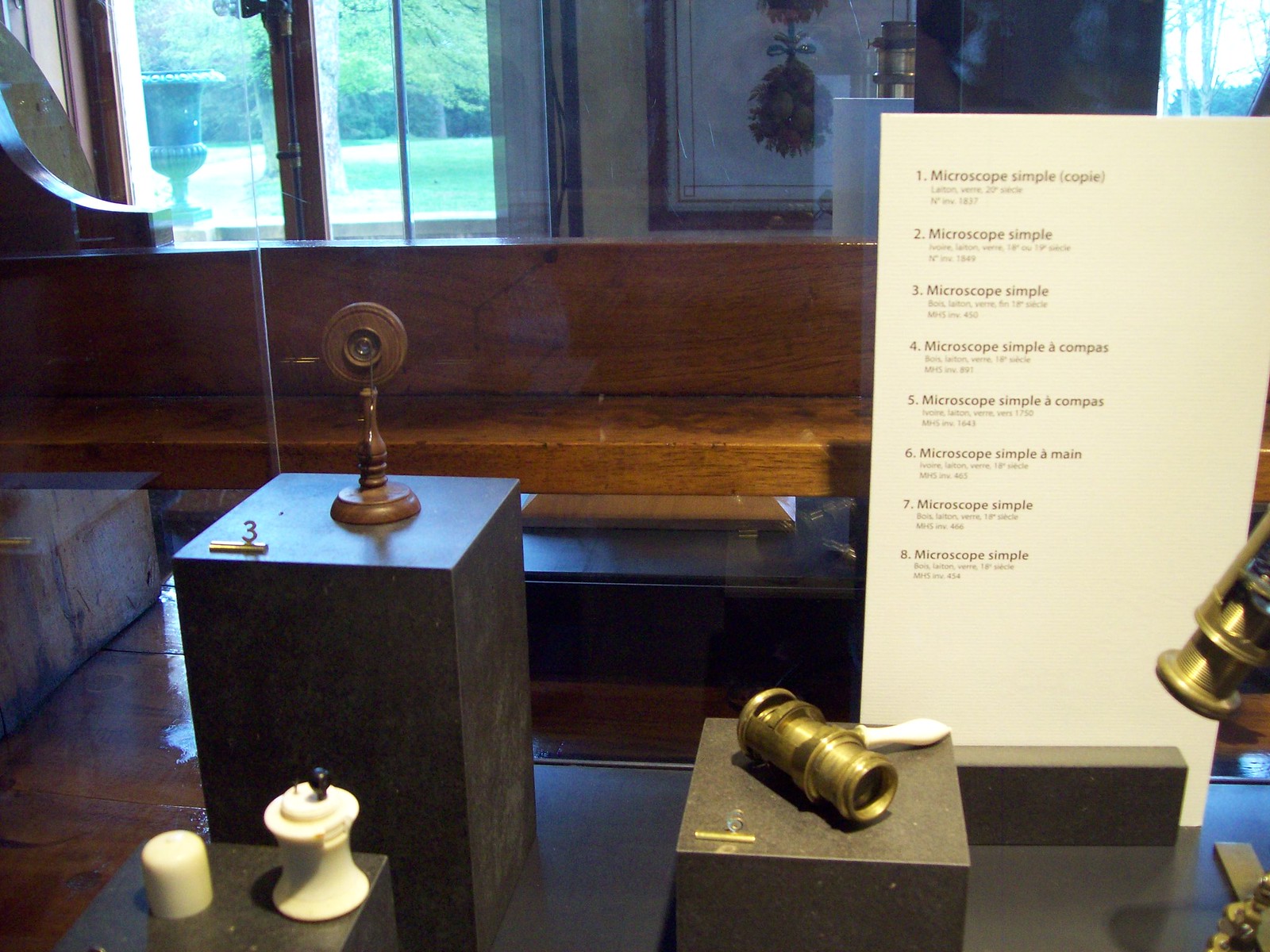This indoor color photograph captures a museum display case showcasing various pieces of early microscope technology perched on black pedestals. Dominating the lower left of the image is a lens, part of a white, curved, cone-shaped structure, while the lower right foreground is highlighted by a cylindrical lens encased in shiny brass. Central to the display, slightly left of center, is a notable lens mounted on a wooden stand. Each of these elements is meticulously placed on black modular stands, which a previous observer likened to granite boxes. In the background on the left side, a placard provides detailed descriptions of the eight microscope samples, although only three of the samples are clearly visible in this shot. Through the glass of the display case, a wooden bench and greenery outside the museum's window can be discerned, adding depth to the scene. The integration of historical artifacts and descriptive elements paints a comprehensive picture of the intricacies of early microscope technology.